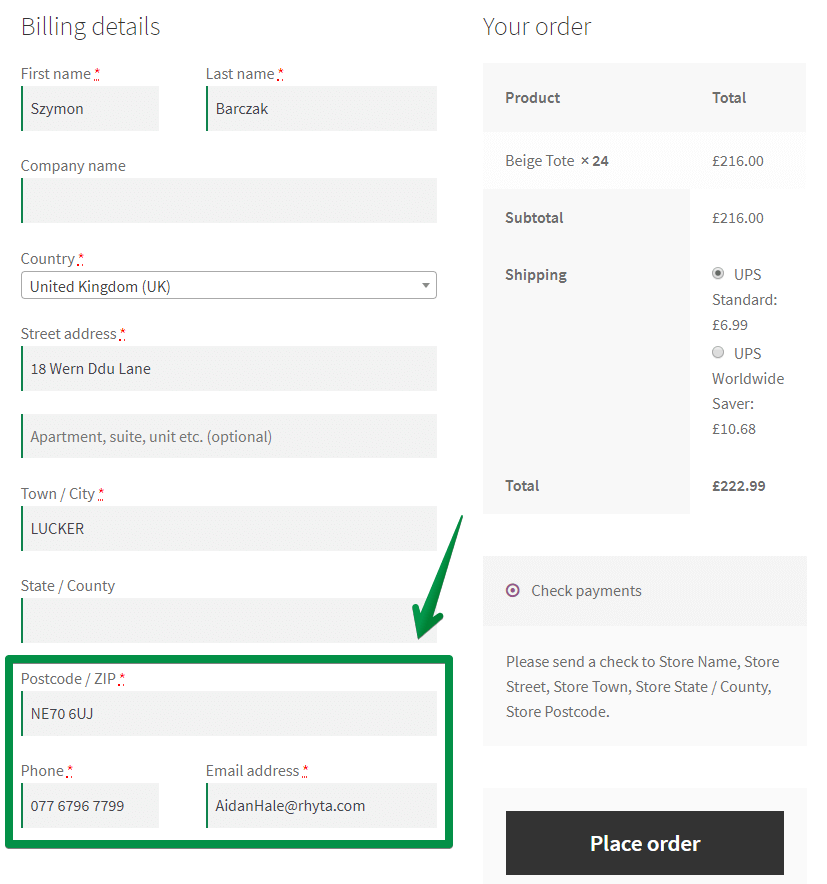This is a detailed screenshot of an online checkout page with a clean white background. At the top of the image, the page is dominated by black and white text. On the left side, the heading "Billing Details" is prominently displayed in black text. Below the heading are various text fields for user information, many of which are marked with red asterisks indicating mandatory fields.

The text fields include:
- First Name (marked with a red asterisk) filled with "Seisminbazak"
- Last Name (marked with a red asterisk) also filled with "Seisminbazak"
- Company Name (optional and remains blank)
- Country (marked with a red asterisk) listed as "United Kingdom"
- Street Address (marked with a red asterisk) filled with "18 Warren DDU Lane"
- Apartment, Suite, Unit (optional and left blank)
- Town/City listed as "Lucker"
- State/Country (field is empty but indicated with a green arrow)

The postcode/zip field is marked with a red asterisk and filled with "NE70 6UJ". Below this are additional fields for phone number (marked with a red asterisk) and email address.

On the right side of the screen, under the heading "Your Order," details are provided for products and their costs:
- "Beige Totes x 24" costs 216 pounds
- Subtotal: 216 pounds
- Shipping options:
  - UPS Standard for 6.99 pounds (selected)
  - UPS Worldwide Saver for 10.68 pounds (not selected)

The total amount due is 222.99 pounds.

At the bottom, the payment method is indicated as "Check Payments" with a small purple mark. The text in gray specifies instructions: "Please send a check to Store Name, Store Street, Store Town, Store State/County, Store Postcode." Finally, a gray and white "Place Order" button is present at the bottom of the page.